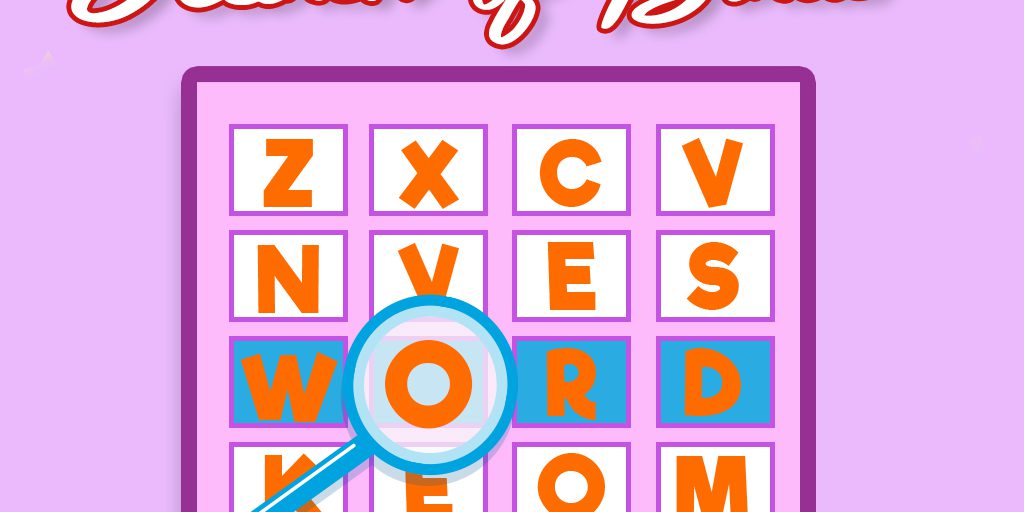In this captivating word game image, a magnifying glass hovers over the letter 'O' at the center, highlighting its significance in forming a word. The grid is filled with a selection of letters: Z, N, W, K, X, C, V, V, E, S, O, R, D, E, and O, each arranged in a seemingly random pattern. The visual palette features vivid hues including deep purple, bright orange, crisp white, and bold red, adding a vibrant contrast to the scene. The intricate details and color choices draw attention to the puzzle, inviting viewers to engage and find the hidden words.